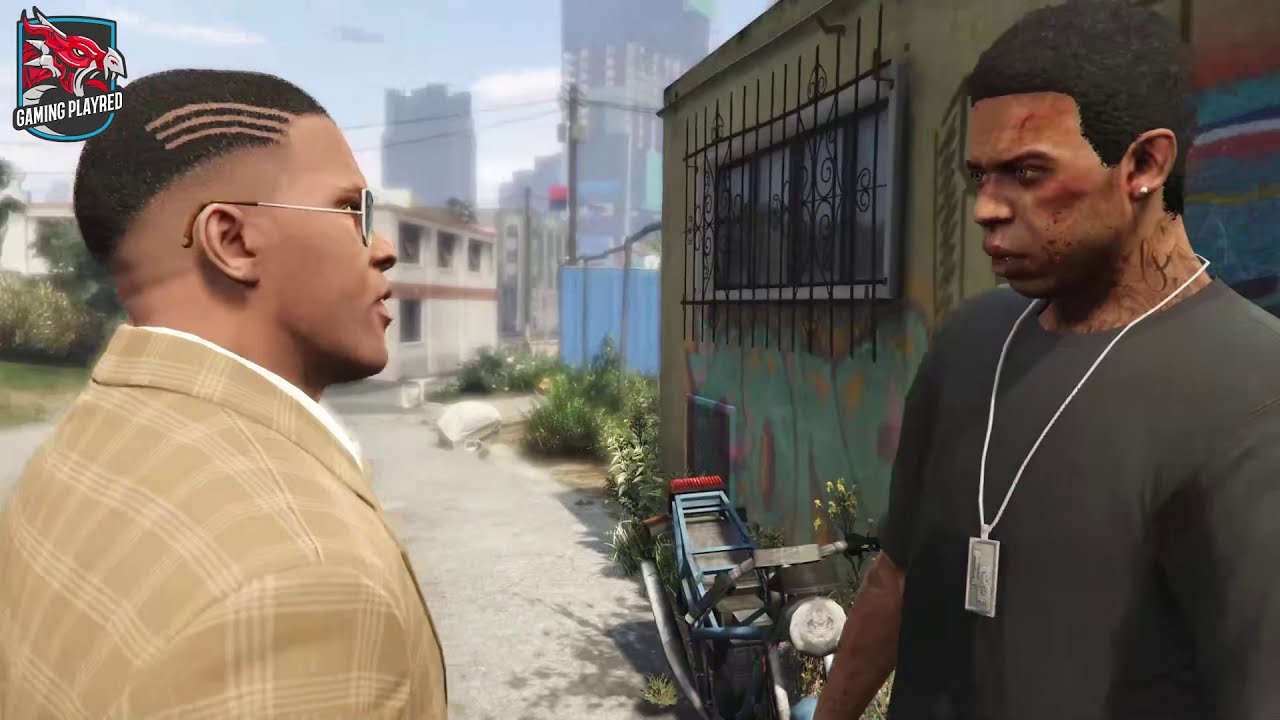This image appears to be a screenshot from a video game, featuring two dark-skinned male characters who seem to be engaged in a serious conversation in an urban, somewhat rundown setting. In the upper left corner is a patch with a fierce, screaming dragon-like face, complete with sharp teeth and a red tongue. Below the dragon, it says "Gaming Play Red" in white lettering.

The man on the left is dressed in a beige plaid sport jacket with white striping over a white collared shirt and is wearing silver aviator sunglasses. His dark hair includes three parallel stripes shaved into it, adding a stylish touch. He appears to be looking curiously at the other character.

The man on the right has very dark skin and an intimidating demeanor, resembling a cartoonish or zombie-like figure. His face is battered with cuts and scratches, and he has a visible scar on his forehead. He’s wearing a dark grey short-sleeved shirt, a large silver chain with a rectangular pendant around his neck, and possibly a pearl earring. He stands near a green trailer home covered in graffiti, with black metal bars over its windows and a blue moped missing its seat nearby.

The backdrop includes a mix of small building structures and tall buildings against a hazy sky, highlighting the gritty, urban environment of the scene.